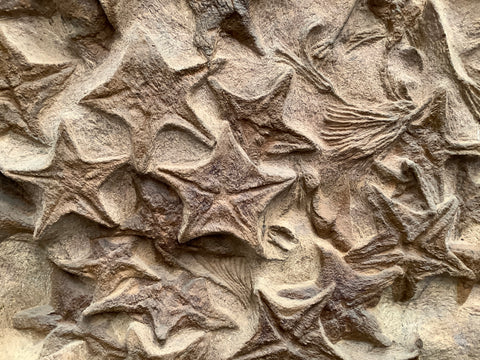This detailed color photograph captures a fascinating archaeological find – a large slab of beige to sandy brown fossilized marine life from Morocco. Primarily consisting of crinoid and starfish fossils, this photograph showcases a close-up section of what might be a larger fossil measuring approximately three to four feet long, two feet wide, and about six to eight inches thick. A central cluster of around a dozen five-pointed starfish fossils stands out, their darker brown coloration contrasting with the lighter sandy background. The starfish display characteristic indentations, with radiating lines extending from their centers to the tips of their arms. Embedded alongside the starfish are other faint remnants of marine life, adding to the textured, ancient feel of the stone. This particular fossil, part of a well-known study area in Morocco, is similar to those sold by specialized companies for significant amounts, highlighting its value and rarity.